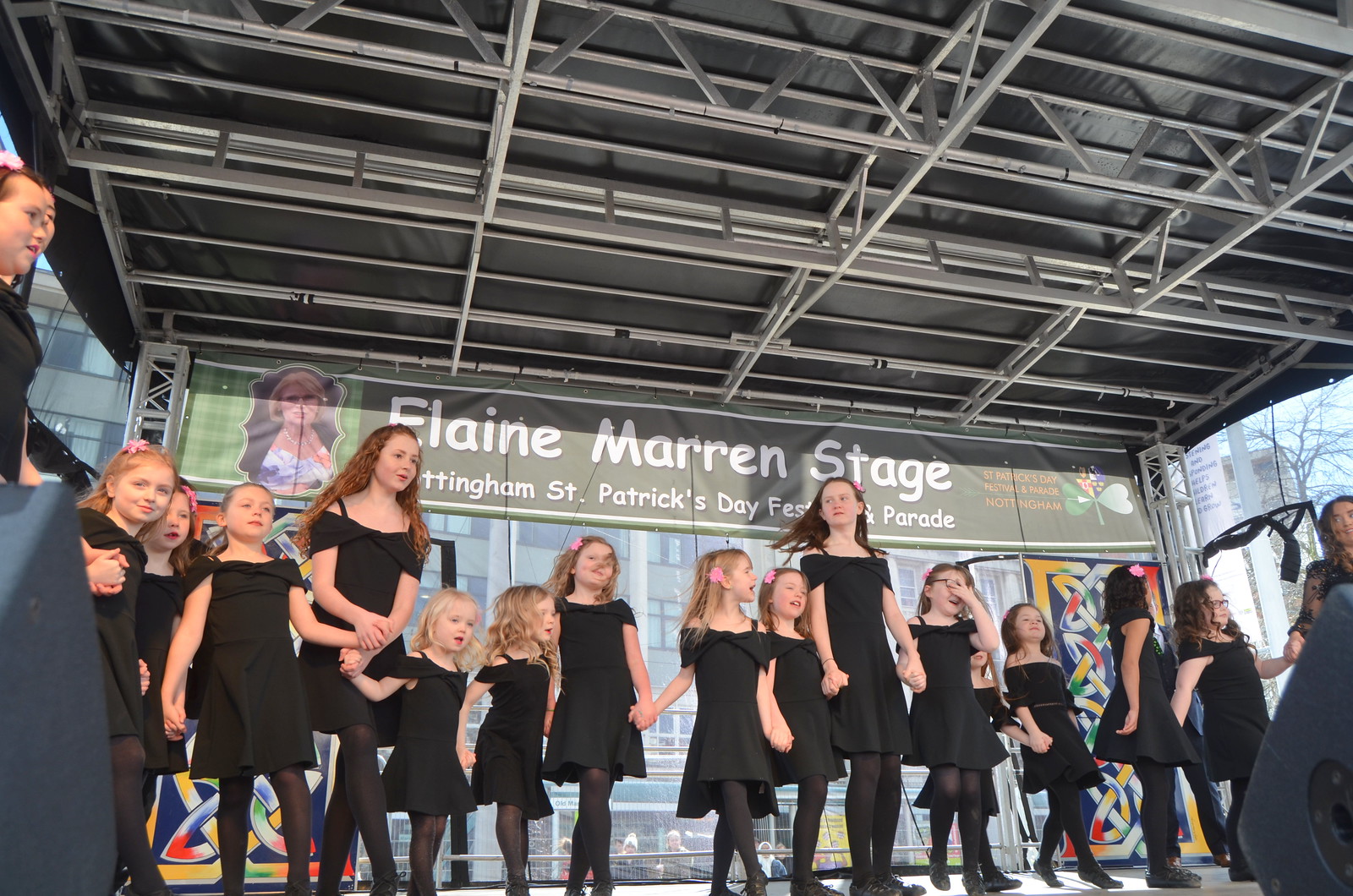In this vibrant color photograph, a lineup of more than a dozen girls, ranging from toddlers to teenagers, are captured mid-performance at the Elaine Marin Stage. The girls, all dressed uniformly in black dresses paired with black stockings, are holding hands in a single row, suggesting they are part of a dance troupe. Above their heads, a banner stretches across the stage, displaying "Elaine Marin Stage" in bold white lettering. Below this, it reads "Nottingham St. Patrick's Day Festival Parade" with a picture of a woman, likely Elaine Marin, on the left side of the banner and a green shamrock on the right, hinting at an Irish cultural theme. The stage is sheltered by a black, aluminum-framed covering, and the photo is taken during the daytime. The dancers' joyous expressions suggest they have just finished an energetic performance, akin to a Riverdance, and are possibly taking a bow amidst a festive atmosphere. A building is visible in the distant background, further situating the event in an outdoor, communal setting.